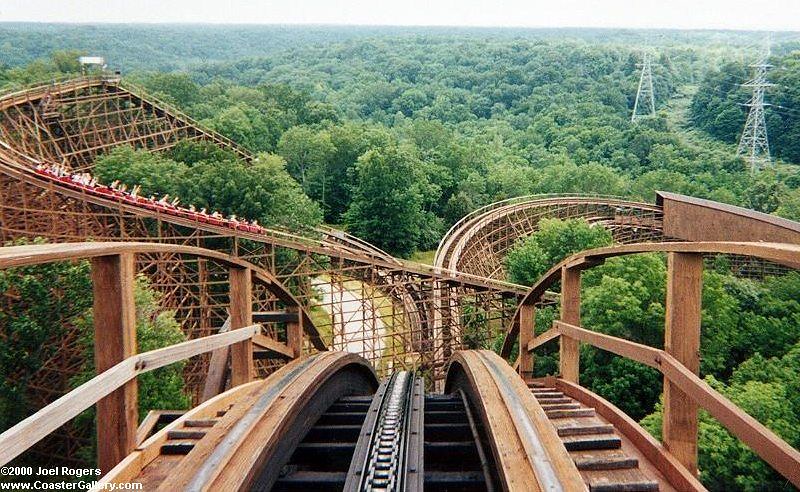Captured from the peak of a classic wooden roller coaster, this photograph by Joel Rogers (copyright 2000, www.coastergallery.com) immerses viewers in the thrilling moment right before the descent. The robust, interlaced wooden structure of the coaster dominates the scene, its intricate framework of timber towering against a backdrop of dense, verdant forest. The metal tracks, framed perfectly in the image, showcase a dramatic right-hand turn leading into a tunnel.

Emerging from the tunnel, the roller coaster tracks rise sharply before plunging again, embodying the anticipation and excitement of the ride. In the distance, a section of the roller coaster reveals a group of passengers with their arms raised in exhilaration. Below the coaster, a small walking trail winds through the sea of trees, while telephone poles and power lines subtly intersect the landscape, hinting at the encroachment of civilization. This evocative shot, brimming with detail, perfectly captures the essence of a thrilling ride amidst nature’s expanse.